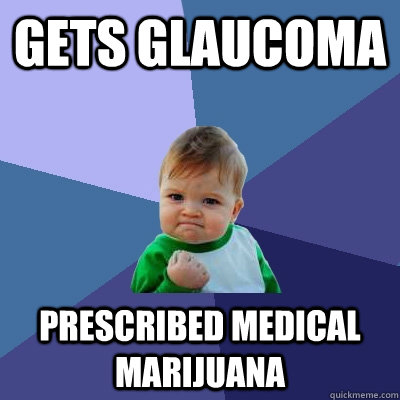This image is a meme featuring a muscular, shirtless white male with a bald head and a gray and black beard and mustache. A small circular tattoo can be seen on one of his biceps. He is wearing only thong-style underwear, resembling a Speedo, and is positioned either sitting, kneeling, or crouching on a bed, straddling a small round pillow that is black with a white stripe. The bed itself is covered with a camouflage-patterned comforter in shades of red, gray, black, and white. Behind him, black pillows with white stripes are arranged against a medium-dark brown headboard. The background wall is dark blue, and at the bottom center of the image, white uppercase text spells out "HAI."